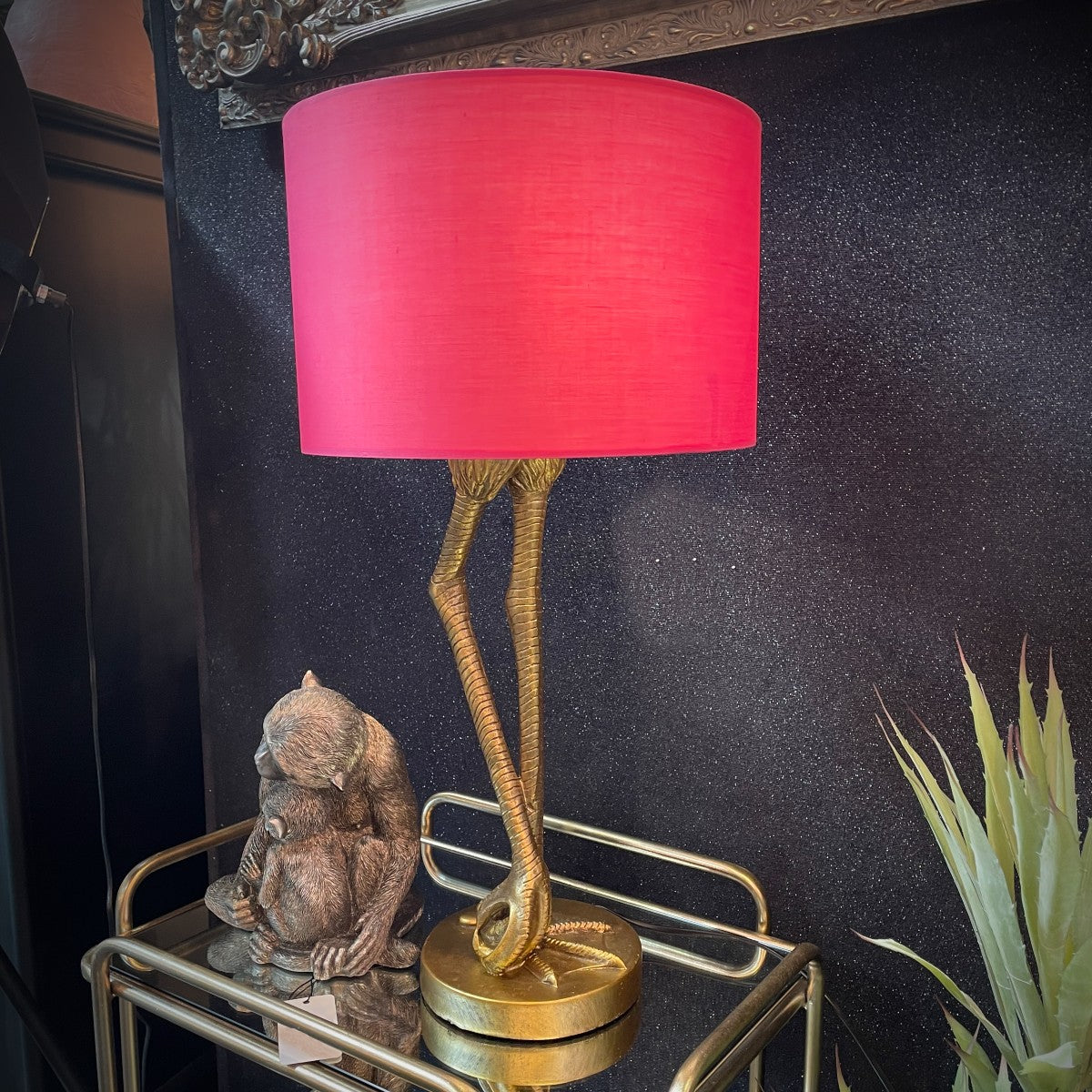The photograph captures an elegantly simplistic scene centered around a unique lamp and its surroundings. Positioned on a small, reflective storage table with a gold frame, the lamp features a bright fuchsia pink, cylindrical lampshade perched atop two long, golden stork-like legs. One of the legs is bent at the knee, and both stand on a round golden base. Accompanying the lamp on the table is a bronze statue depicting a monkey cradling a baby monkey tenderly. The backdrop is a glittery textured black wall adorned with various white specks, adding a touch of sparkle to the scene. In the bottom right corner, the tall, notched leaves of an aloe plant peek into the frame, adding a natural element to the composition. At the top center of the image, a picture frame is faintly visible, hinting at additional decor above the main subjects.